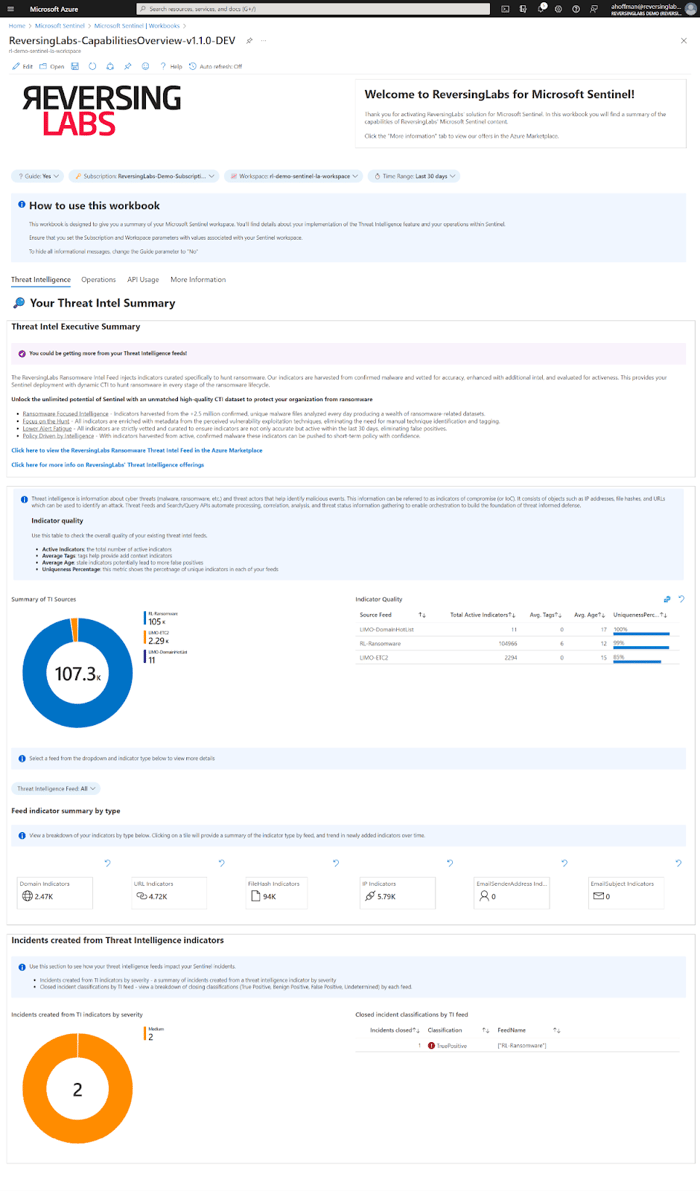In this image, a highly zoomed-out view of the Reversing Labs website is displayed. The title "Reversing Labs" is visible with "Reversing" in black and "Labs" in red, which stands out prominently due to the extremely small text throughout the rest of the page. At the top of the image, the background is black and features a search bar centered in this strip. Below the search bar, there is a series of text sections, some highlighted in light blue, while others have a plain white background.

Toward the middle of the image, there is a blue circle with "107.3" written in the center, accompanied by a small orange line at its top. To the right of this circle, there are four informational fields. As we move further down, more categories and sections continue, extending to the bottom of the image.

At the bottom, an orange circle with the number "2" in the center is visible, featuring a slight white sliver at its top. The predominant background color of the page is white, however, specific pieces of information and titles are highlighted with either light blue or light gray backgrounds, adding contrast and organization to the visual presentation.